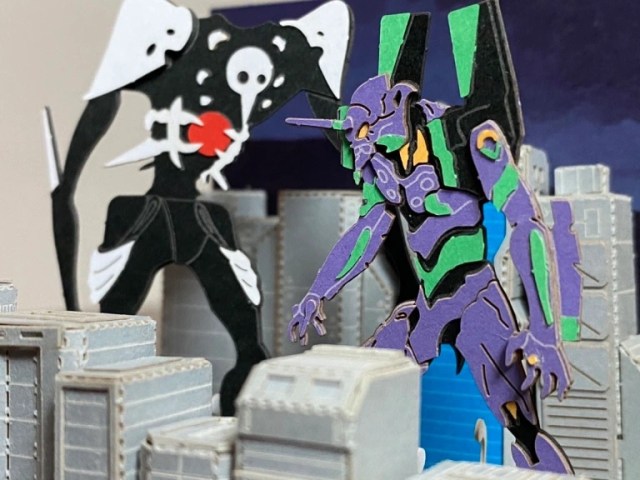The image depicts a meticulously crafted scene featuring two science fiction mechas engaging in battle amid a detailed miniature cityscape. The foreground showcases a predominantly purple mecha with design elements reminiscent of the anime "Neon Genesis Evangelion." This mecha has an intricate design, featuring a small elephant-like head with gold eyes, accented with green on the torso, and wearing impressive armor. Its opponent, situated further back in the scene, is a striking black mecha with a white face, exhibiting a bird-like head with a pointed beak and a red circular feature on its chest. The backdrop of the scene includes carefully constructed buildings, resembling a toy city, possibly made from materials like styrofoam. The attention to detail in both the mechas and the cityscape suggests a vivid depiction of an impending sci-fi battle.